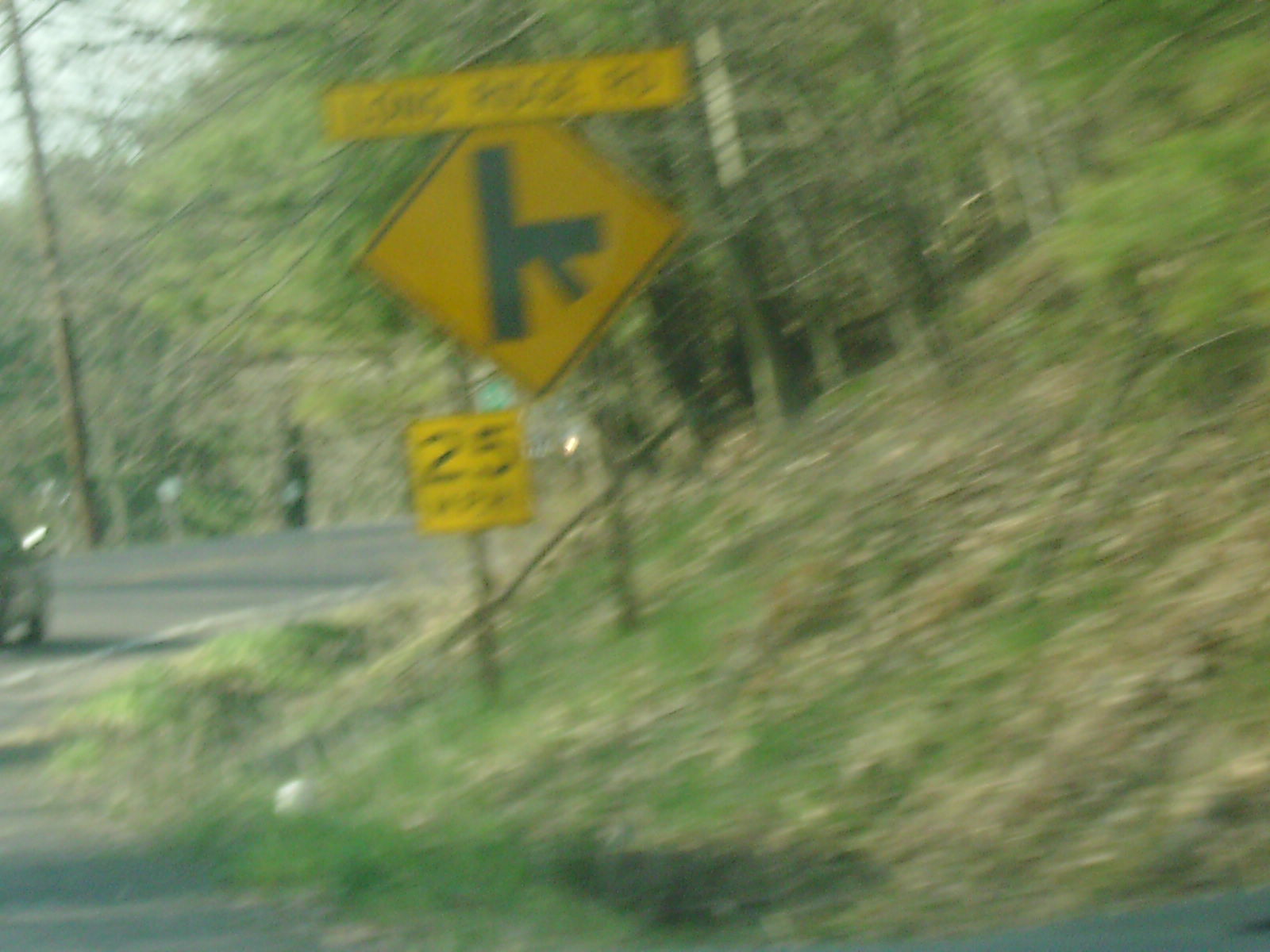The image depicts a cluster of three road signs set against a grassy, sloped verge adorned with trees. The signs, all yellow with black borders, provide essential warnings and instructions for road users. 

The primary sign is square-shaped and prominently displays "25 KPH," indicating a speed limit of 25 kilometers per hour. The number "25" is written in large, bold letters above the smaller abbreviation "KPH."

Just below this sign is a diamond-shaped warning sign that alerts drivers to a road junction ahead, an essential cautionary symbol for motorists.

Mounted atop the diamond sign is a rectangular sign with indecipherable text, whose specific warning or instruction remains unclear.

The backdrop includes a road, partly visible on the left side of the frame, where a vehicle can be seen navigating around a bend. The scene is captured in daylight and is well-lit, enhancing the visibility and clarity of the signs and surrounding landscape.